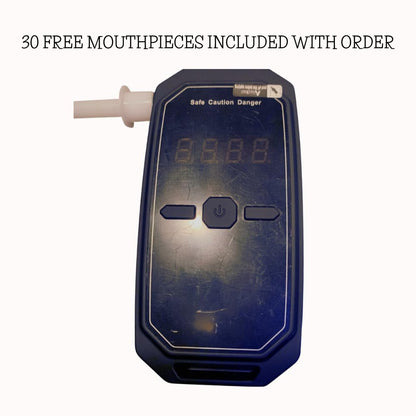This photograph features a somewhat worn-looking breathalyzer device at its center, positioned against a stark white backdrop. Resembling a remote control or a small gadget with squared-off corners, the mostly black device features three buttons: a central power button flanked by two arrow-shaped buttons. Above the buttons is a digital screen, currently turned off, that would typically display numerical readings. Directly above the screen, white text labels the sections "safe," "caution," and "danger." Extending from the top-left of the device is a white breathing tube, which users blow into to measure their alcohol content. Notably, the device's surface is visibly scratched, hinting at prior use, especially as light reflects off the damaged areas. Superimposed black text above the photograph states "30 free mouthpieces included with order," suggesting this image is likely an advertisement for the breathalyzer, perhaps from an online shop.